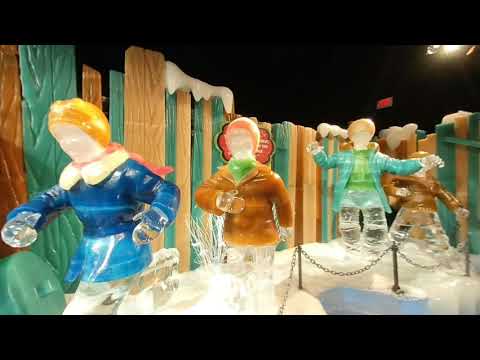This image depicts a close-up view of what seems to be a winter-themed display, likely a Christmas setup at a department store or mall. The scene features four figurines made of transparent material, resembling glass or ice, detailed with vivid clothing. At the front is a girl with blonde hair, dressed in a blue jacket with a white fur collar, and a yellow and orange ski cap. Behind her is a boy wearing a brown and tan coat, a green scarf, and an orange ski cap. The third figure is a larger boy in a light blue jacket over a green shirt. The last character, positioned further back, wears a brown jacket. They are all positioned as though frolicking through snow, with their translucent legs accentuating the icy theme. The scene is set against a brown and green snow-covered fence, forming a winter backdrop. The entire display appears to sit on a tabletop under a stark black sky with overhead lighting, enhancing the ethereal, frozen ambiance of the composition.